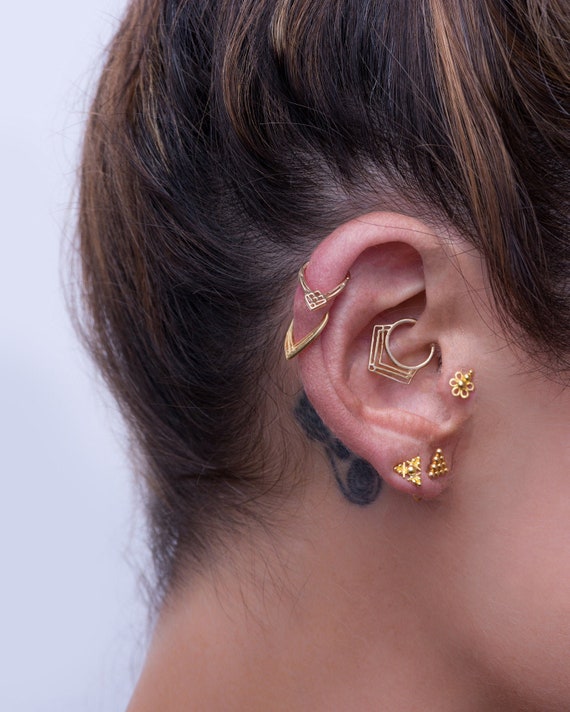This detailed photograph features the side profile of a woman’s head against a grayish light blue background. The focal point is her ear, adorned with multiple pieces of golden jewelry. She has pale to tan skin and her hair, styled in an updo, is dark brown at the roots transitioning to lighter brown with hints of light brown highlights towards the ends. Behind her ear, there is a black tattoo.

Her ear displays an array of intricate jewelry: two rings on the outer lobe, two earrings in the fleshy part of the lobe, and a flower-shaped stud on the small, rounded front part of the ear. Additionally, the middle cartilage bears two rings. The jewelry includes various V-shaped pieces, loops, and patterns including floral and triangular shapes, all with a golden appearance. The photograph captures part of her cheek near the ear and the hair on the back of her neck, emphasizing the detailed and visually rich adornments of her ear.